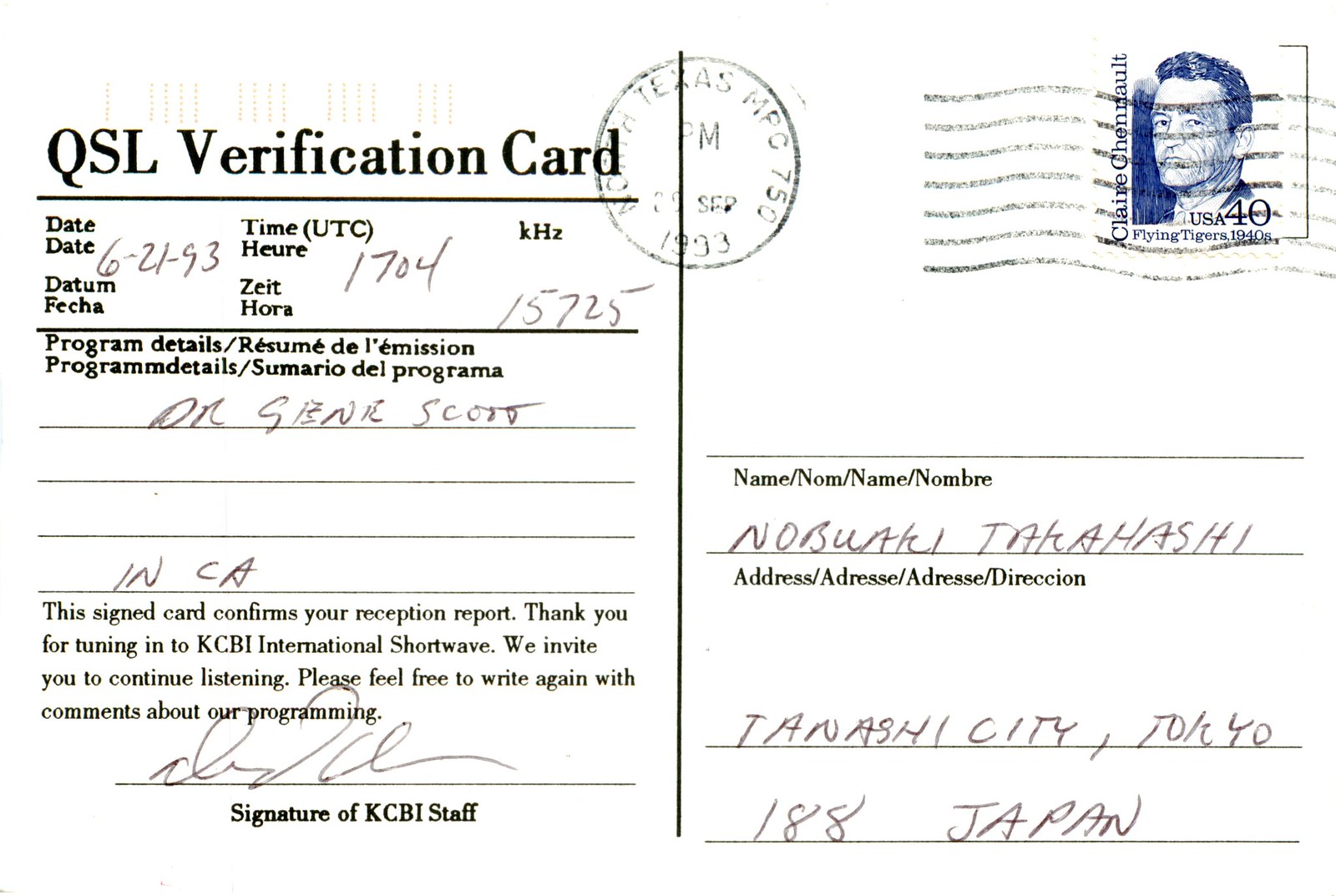The image is of a predominantly white postcard used as a QSL verification card, often sent to confirm the reception of a broadcast station. It is divided vertically into two sections by a solid black line. On the left side, in black text, it reads "QSL Verification Card" and is followed by a horizontal black line. Beneath this, the card details the date as "6-21-93," the time as "17:04," and the frequency as "KHz 15725." Another horizontal black line separates this from the sections below that contain "Program Details." Handwritten beneath this section are the names "Orseen Scott, NCA." Printed in black text, it reads, "This signed card confirms your reception report. Thank you for tuning in."

On the top right corner of the postcard is a blue stamp featuring the face of Claire Chennault and labeled "USA 40 Flying Tigers 1940s," overlaid with faded stamp markings. The card further invites the recipient to continue listening and offers an invitation to write back with comments about the programming. The closing section includes a signature from KCBI staff with the printed name "Nobuaki Takahashi" and the address "Tanashi City, Tokyo 188, Japan." Also mentioned is a more detailed thank-you message for tuning in to KCBI International Shortwave.